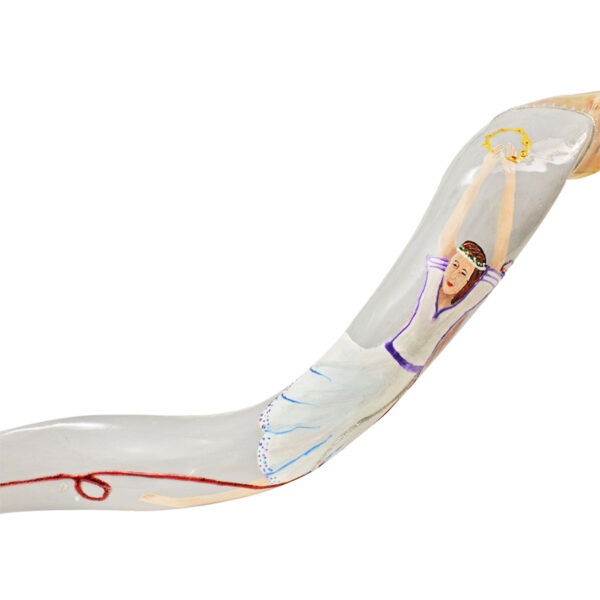On a pure white background, there is an image of a curved, cylindrical wooden object that has been isolated, possibly through Photoshop, with careful detailing in white paint. The object features a depiction of a woman dressed in a white dress with three blue stripes around the half-sleeves and a blue band cinched at her waist. She has brown to black hair adorned with a white headband, and her lips are vividly painted red. The woman is depicted with her hands raised above her head, holding a golden tambourine, which might suggest she is dancing, possibly in a band or participating in a ritual ceremony. She exudes an aura of joy and fun. Running down the object is a red ribbon that loops near her feet and continues off the edge of the image. The top of the cylindrical object shows some natural brown wood exposed.